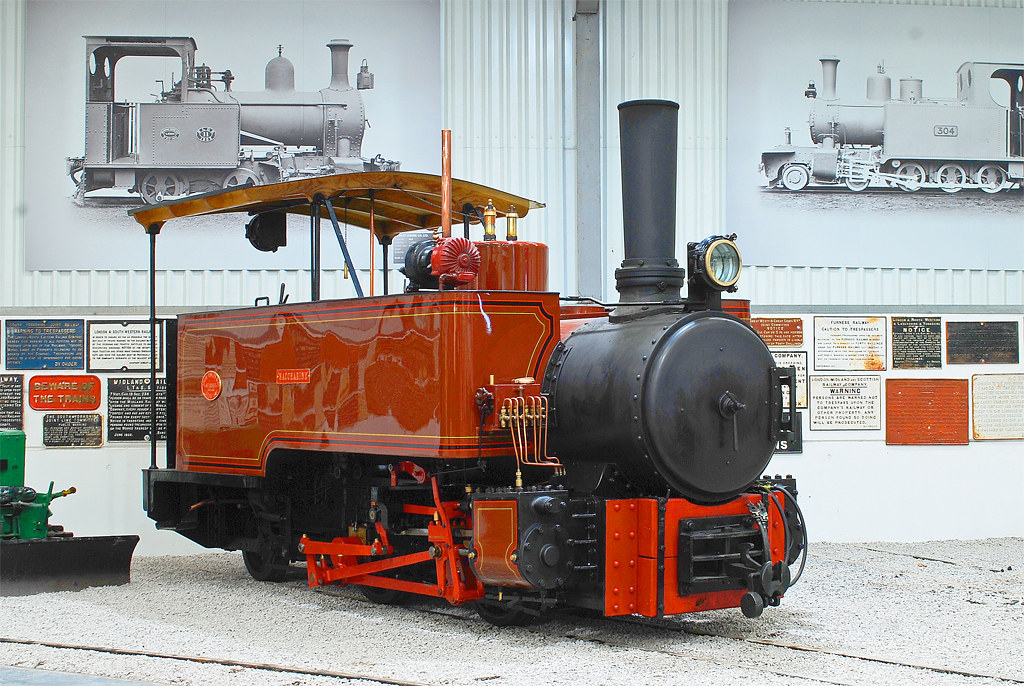This photograph showcases a beautifully detailed, miniature steam locomotive, predominantly painted in red with a black boiler and chimney, highlighted with brass whistles and decorative gold detailing. The engine, which appears to be in immaculate condition with a glossy finish, prominently occupies the center of the image. It features a curved wooden roof, a connector on the front for additional cars, and meticulously crafted black wheels with red mechanisms for turning them. 

The background is adorned with a variety of plaques and signs, including black and white photos and diagrams of full-size engines, likely switch engines used for tasks such as maneuvering cars within rail yards or smaller-scale operations like hauling sugar cane in the Caribbean. These photographs and other train-related memorabilia, such as colored plates with unreadable fonts and signage like a red "beware of trains" notice, suggest the setting is a museum dedicated to preserving railway history. The locomotive is displayed on a small, gray track area, set against a backdrop of clean white walls and floor, enhancing the exhibit's organized and educational ambiance.